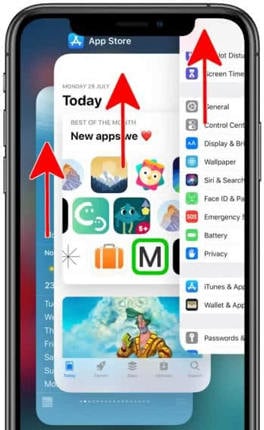This image showcases a cell phone, highlighting both its front and side views. The phone's screen displays the App Store, albeit in a slightly blurry manner with multiple icons visible. At the top, the screen reads "Today" with a red arrow pointing upwards, emphasizing the recent activity on the phone. Beneath this, the weather application is prominently shown, also marked with a red upward arrow, indicating it was the first app accessed. Additionally, numerous settings icons are visible, suggesting the user recently navigated their settings. Another red arrow signifies this activity. The screen also reveals the phone's wallpaper, which is visible when no apps or websites are open. The bottom part of the phone is not visible, but the physical buttons are: three on the left side and a single button on the right side, which functions to power the phone on or off and to capture still pictures.